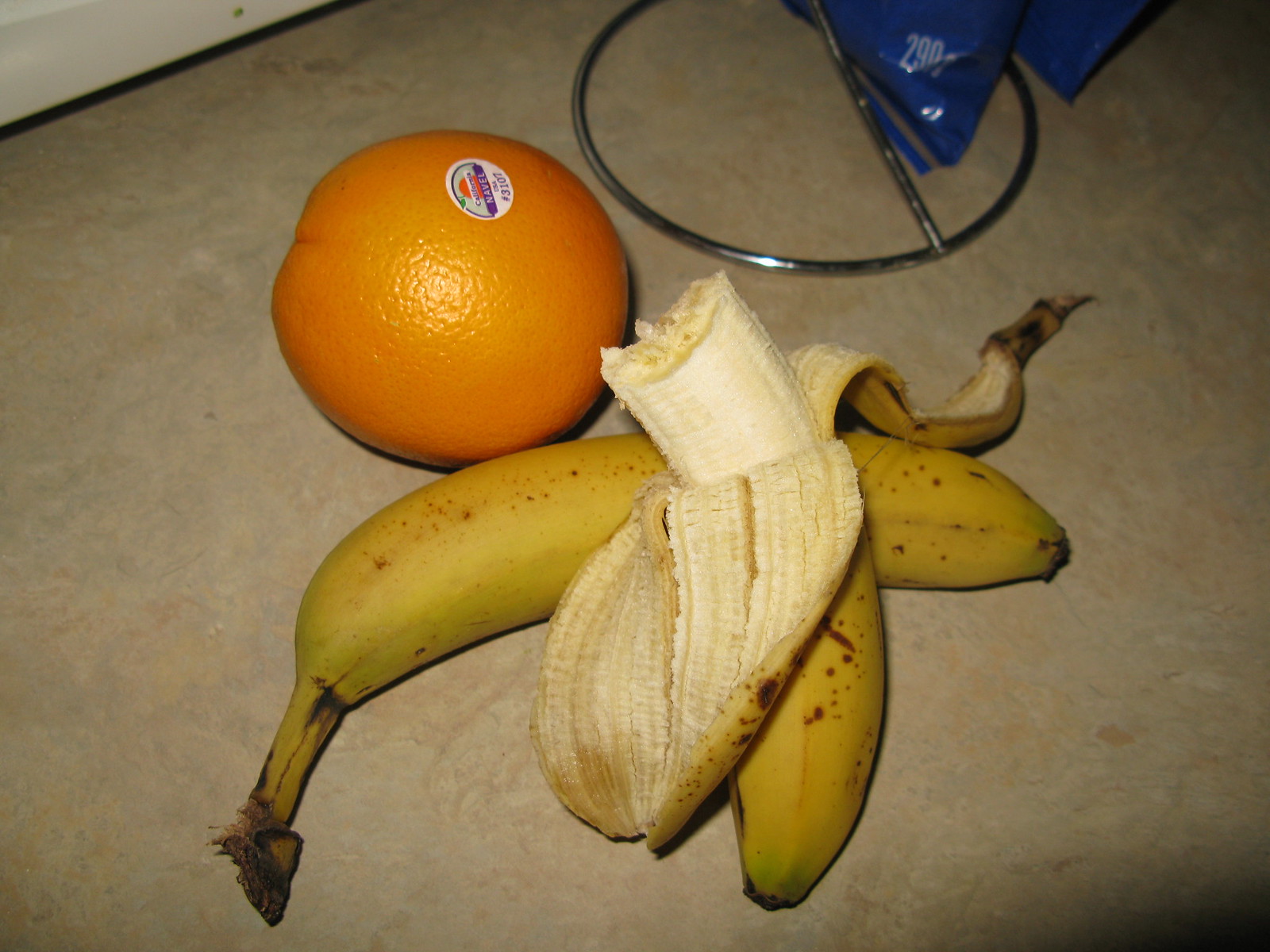A detailed image showcases a variety of items lying on a beige carpet, often used in high-traffic areas. Central to the scene is an unpeeled orange adorned with a sticker that reads "Navel" along with the serial number 3107. Nearby, a yellow banana with brown spots rests with its stem pointing downward. Draped over this unpeeled banana is a partially peeled one, revealing its eaten, creamy interior. Adjacent to the fruit lies a shiny, steel circular object, accompanied by a blue plastic bag marked with the number 290 at its bottom. The setting appears to be indoors, adding a sense of domestic familiarity to the composition.